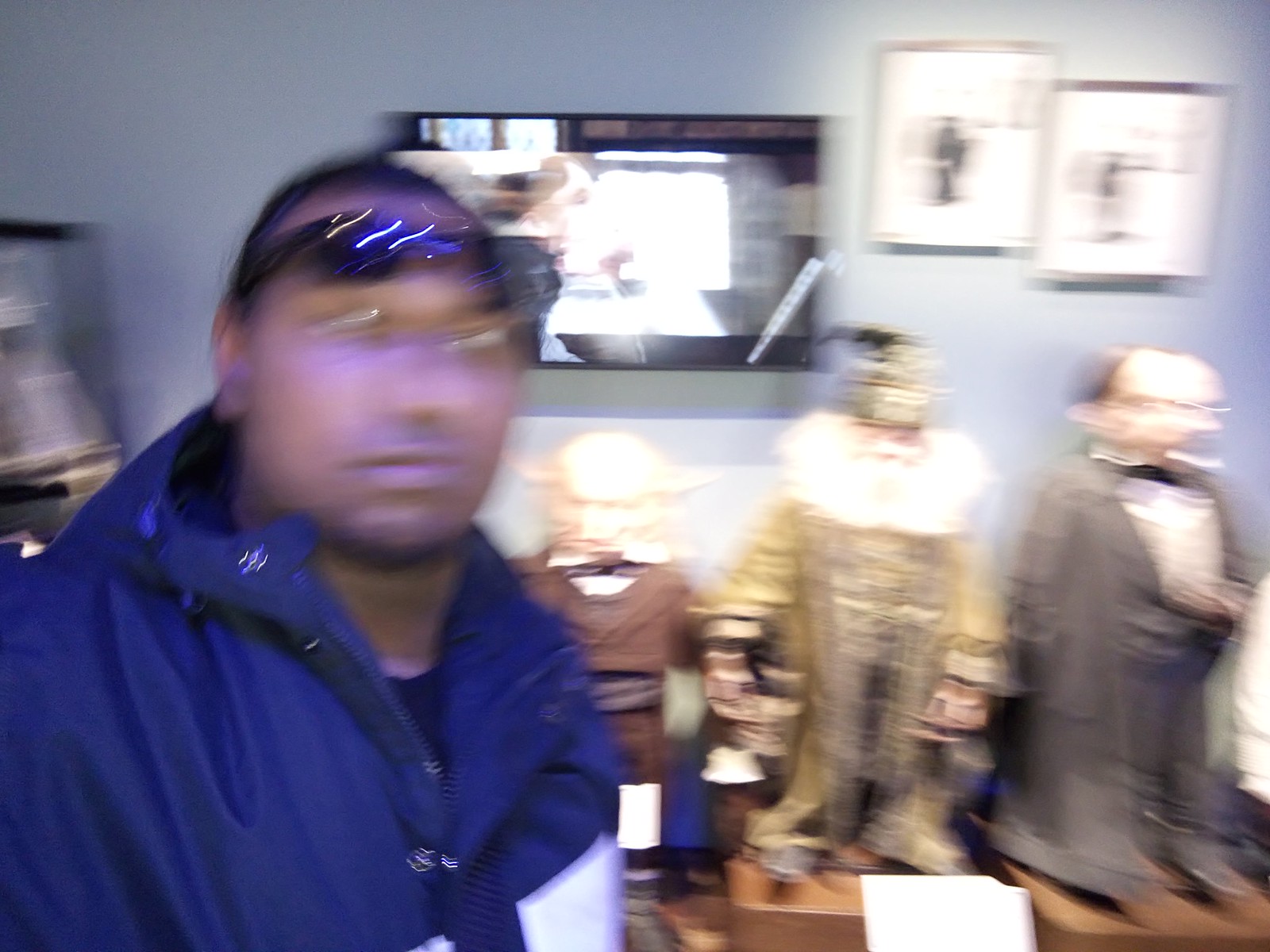In this very blurry image, a black man is positioned in the left foreground, wearing black sunglasses on his forehead and a short hairstyle. He sports a dark blue jacket with white squares or a stripe in the middle. He appears to be glancing to his right. The background features an array of peculiar statues or puppets displayed vertically on a tan, wooden stand. Three distinct figures are identifiable: one in brown with large ears, a central one in a goldish outfit resembling a wizard, and another in gray. Additionally, there are blurry picture frames, a small flat-screen TV, and a light gray wall completing the scene. The overall composition and multiple elements in the image are heavily obscured by the blur.